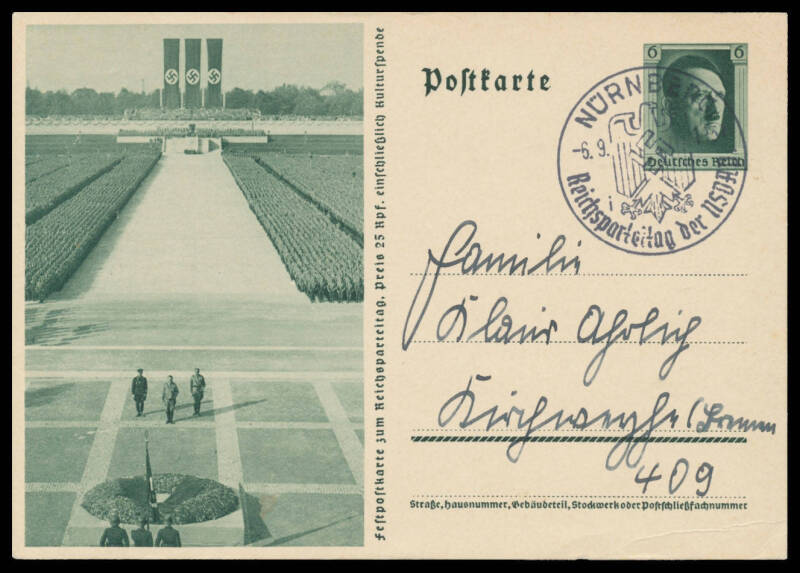This photograph showcases an old postcard from the 1930s, set against a black background. The postcard features a Nazi Germany scene on the left side, capturing a black-and-white image with a greenish tone. Adolf Hitler stands prominently at the center of a stage, flanked by two generals, addressing a vast assembly of soldiers standing at attention. In the foreground, you can see a pathway lined with soldiers on both sides, leading up to three large, vertically-hung Nazi flags displaying black swastikas on white circles. Beyond the flags are trees and an overcast sky. The right side of the postcard shows a handwritten German address, topped by a stamp featuring Adolf Hitler's portrait, marked with the number '66' and postmarked from Nuremberg. The stamp also includes Nazi insignia, and the postcard itself is in remarkably good condition, save for a slight wrinkle in the bottom right corner, preserving a poignant historical artifact.